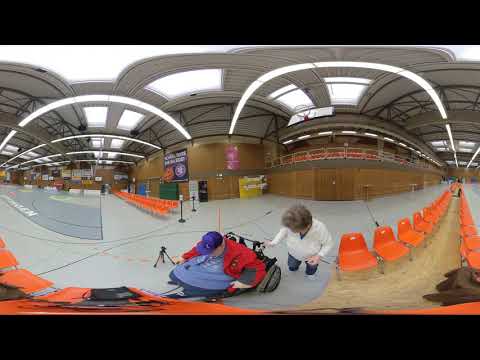The image depicts the interior of a tall, somewhat utilitarian building likely used as a transportation station or gymnasium. This vast, high-ceilinged space, supported by exposed metal beams and illuminated by numerous lights, features plastic chairs with orange seats and metal legs arranged in rows, indicative of a waiting area. In the foreground, an older woman with short gray hair, dressed in a white sweater over a dark top and dark pants, stands behind a man seated in a wheelchair. The man, notable for his larger frame, is wearing a blue shirt, dark pants, an unzipped red jacket, and a blue hat. He appears to be pulling himself forward in the wheelchair. Beside them stands a tripod, and behind them are wooden walls adorned with various signs. The left side of the image hints at a floor resembling that of a basketball court. The second story of the building includes a seating area, with several windows allowing light into the spacious interior. Reflective surfaces create a mirrored effect, repeating portions of the scene.